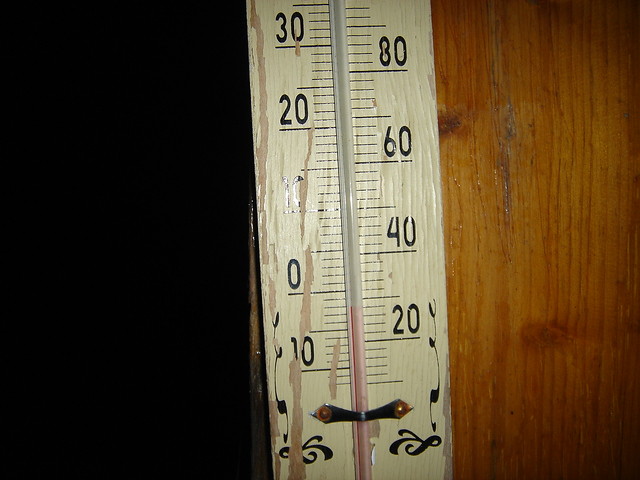In the image, there is an antiquated thermostat featuring dual scales, with Celsius readings on the left side and Fahrenheit on the right. The device, made from what appears to be a red mercury-type material, exudes an old-time charm. It is mounted on a faded, white-painted surface that displays black markings, now faint and chipped, indicative of its age and wear. The temperature reading is just below 30 degrees Celsius, approximately 28 degrees. The paint on the thermostat is deteriorating, showing cracks that suggest long periods of exposure.

The thermostat is affixed to a brown board, giving a sense of prolonged placement. A shadowy area is visible to the left of the thermostat, leaving the setting—whether indoor or outdoor—ambiguous. This shadow also casts doubt on the accuracy of the temperature reading, hinting at a colder ambient environment.

Intricate scrollwork embellishes the bottom right and left corners of the thermostat, adding a decorative touch. Furthermore, a small brass piece can be seen securing the glass cover in place. The overall scene resonates with a vintage aesthetic and a history of sustained use.